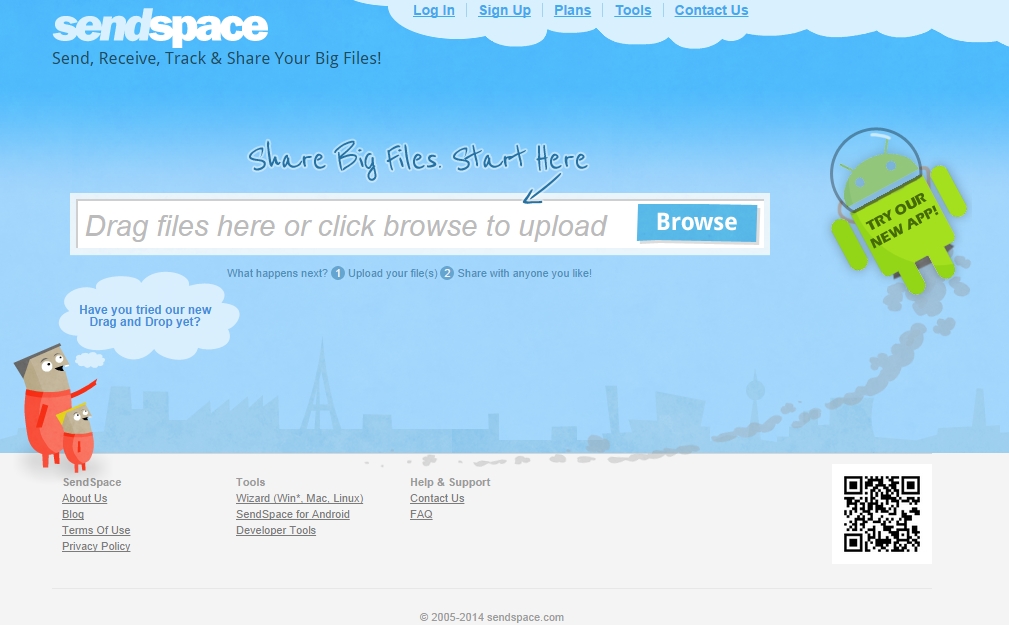This image is a screenshot from the home page of the file-sharing website SendSpace. The background features a soothing sky blue color. Dominating the upper right side, there is a whimsical depiction of a white cloud formation stretching from the center to the upper right corner. Within the central area of this cloud, buttons for various functions like "Login," "Sign Up," "Plans," "Tools," and "Contact Us" are prominently displayed. 

To the left of these buttons, the SendSpace logo is accompanied by the tagline, "Send, receive, track, and share your big files." Directly below this, in the center of the image, bold text commands attention: "Share big files, start here." An arrow extends from this text, pointing to a central box labeled, "Drag files here or click browse to upload." Within this box, a conspicuous blue "Browse" button sits on the right side.

Just beneath this box, on the left side, two cartoon-like characters dressed in red prompt users with the question, "Have you tried our new drag and drop yet?" To their right, an android character clad in an astronaut suit enhances the futuristic theme. Accompanying the astronaut, step-by-step instructions detail the process: "1. Upload your files. 2. Share with anyone you'd like."

At the bottom right corner of the image, a QR code invites further interaction. Conversely, the lower left corner is organized into additional navigational sections for "SendSpace," including "About Us," "Tools," and "Help and Support."